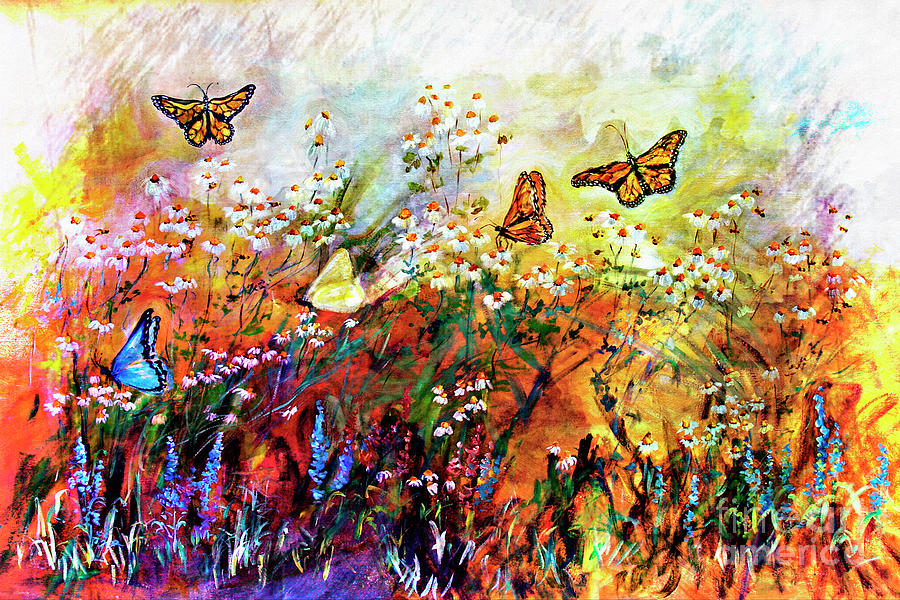This vibrant, oil-painted scene depicts a lively outdoor flower garden, slightly wider than it is tall. The composition bursts with color, ranging from warm hues like yellows, oranges, and reds to cool tones including blues, purples, and teals. The lower terrain of the painting is filled with vertical lines and areas saturated with a rainbow palette of colors. 

Adorning the garden are various plant life and wildflowers, creating an impression of spring. Among the flowers are white petals with orange centers, lavender-like blooms, and thin-petal flowers in shades of pink and red, all accentuated by tall green stalks and grasses. 

Three monarch butterflies prominently flutter around the center-right and upper left of the painting, displaying their distinctive black and orange wings. Additional butterflies, featuring blue and yellow wings, add to the lively atmosphere. The subtle smudgy background, a mix of whites, turquoise, blues, and earthy browns, enhances the sense of a breezy, light-filled day, despite not being overly bright. 

The detailed scene is topped off with a delicate white signature at the bottom right, leaving an indelible mark on this captivating depiction of nature's beauty.